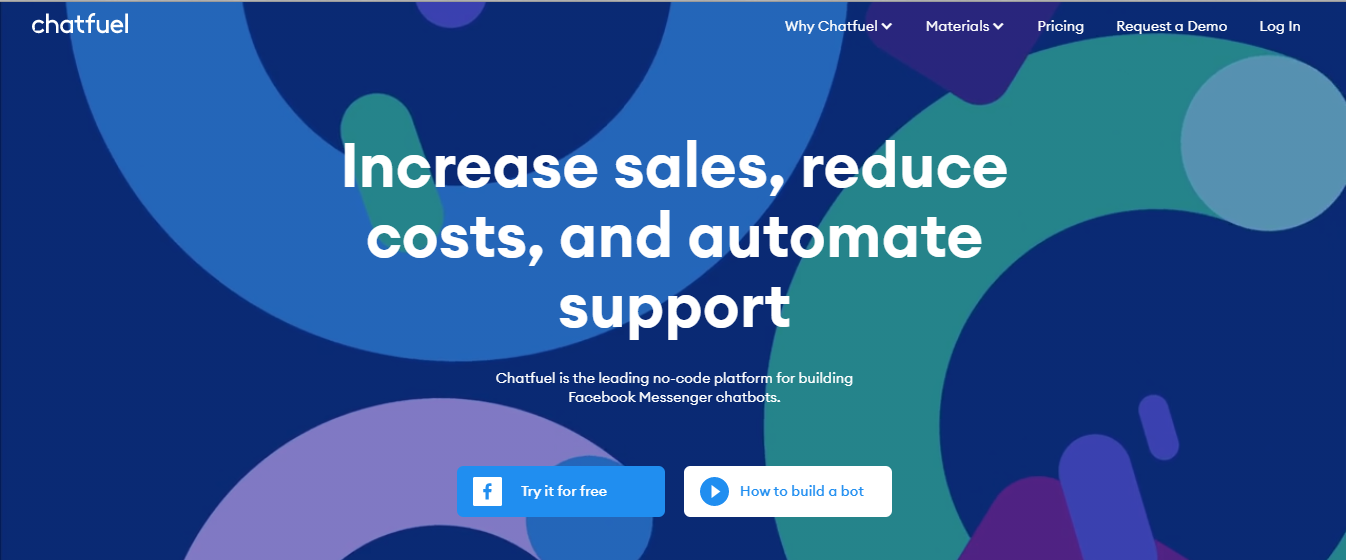The image features a webpage or application interface focused on ChatFuel, characterized by a predominantly blue background adorned with vibrant, colorful half-circle icons in blue, green, and pink hues. 

At the top left corner, white text spells out "ChatFuel." To the right, the navigation menu includes white text links titled, "Why ChatFuel?", "Materials," "Pricing," "Request a Demo," and "Login." 

Dominating the center of the page, large bold text reads, "Increase Sales, Reduce Costs, and Automate Support," showcasing the primary benefits of using the platform. Below this, smaller text further describes the service: "ChatFuel is a leading no-code platform for building Facebook Messenger chatbots."

Towards the bottom, two prominently placed buttons invite user interaction. The first is a blue button with a Facebook logo, labeled "Try it for Free." The second is a white button with blue text that says "How to Build a Bot," featuring a blue circular play icon, suggesting an instructional video link.

The design of the page is clean and straightforward, efficiently conveying the core functionalities and benefits of ChatFuel, while providing clear call-to-action options for users interested in exploring or utilizing the chatbot-building platform.